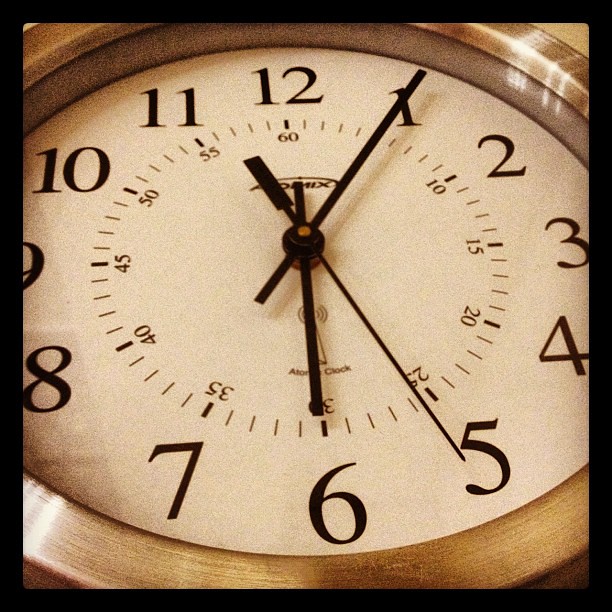This photograph features a close-up image of a round clock with parts of its edges extending beyond the frame, resulting in the 3, 4, and 9 being partially cut off. The clock boasts a brushed silver, antique finish around its casing, which has hints of black paint worn off to give it a vintage look. The clock face is an off-white, cream color with prominent black numbers marking the hours from 1 to 12. Each hour is detailed with smaller lines denoting minute increments, and every fifth-minute interval (5, 10, 15, etc.) is marked with thicker, darker lines. Between these intervals are thinner, lighter lines to indicate each minute. There is a secondary inner circle featuring additional dashes and numbers, likely indicating seconds, with the second hand partially covering the brand name located under the 12. The clock also prominently displays "Atomic Clock" at the bottom. All three hands—the hour, minute, and second—are black, indicating a time of 11:04.